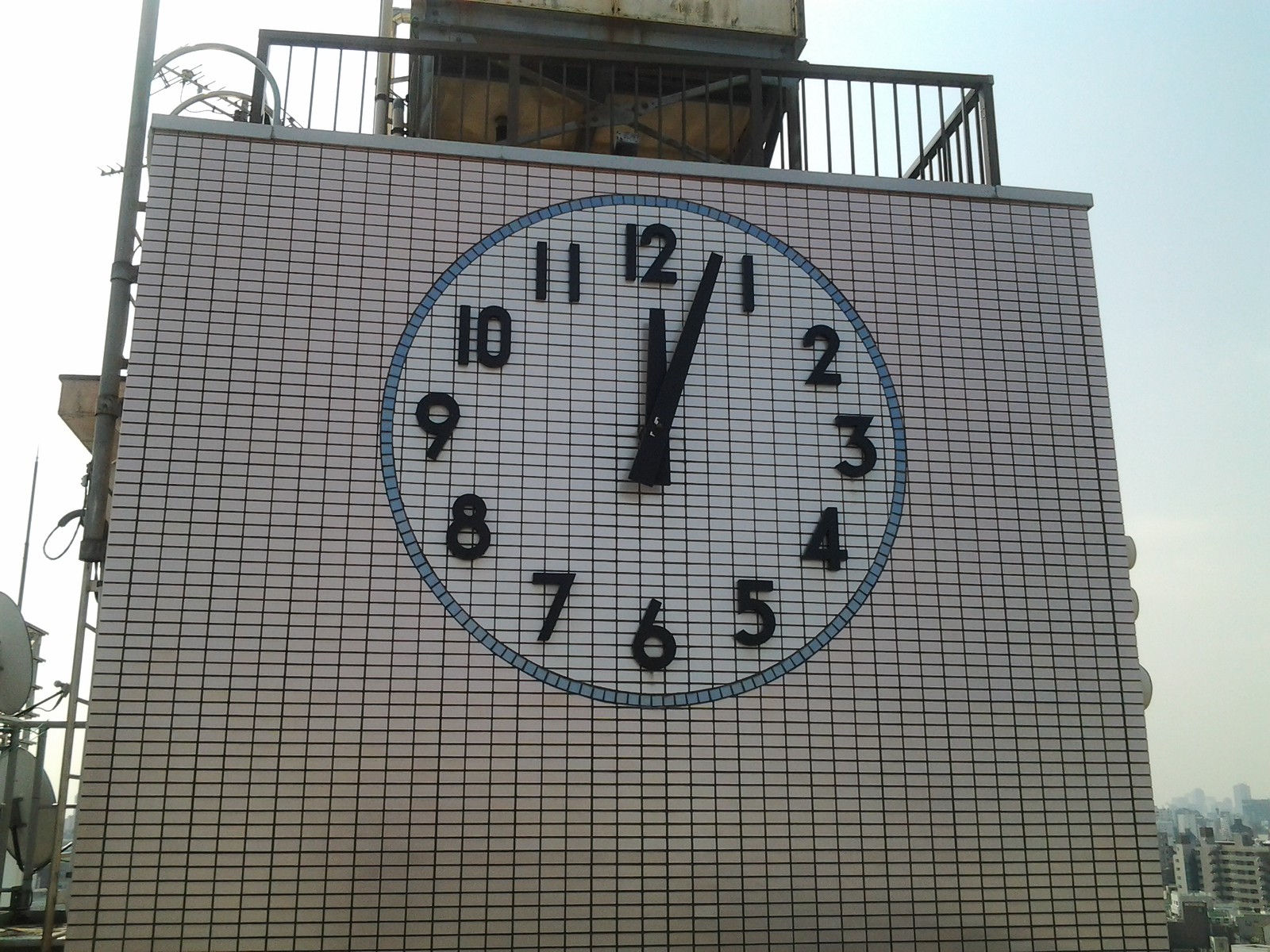This photograph captures an outdoor scene featuring a substantial, peach-colored brick wall adorned with a traditional, non-digital clock at its top center. The clock, embedded into the brickwork, has a white face with cyan blue edges and black, three-dimensional numbers. Its little hand points directly at 12 while the big hand rests between the 3 and 4, indicating around 12:03. The surrounding wall segment featuring the clock is distinctly white brick, contrasting with the predominantly peach-colored surface of the rest of the wall. At the top of the wall, there is a dark gray railing with small cylindrical rods, and a wooden box-like structure extending upward, possibly suggesting the base of a tower, though it is partially cut off. The scene is set in a city during the daytime under a bright, mostly clear sky with patches of cloud.